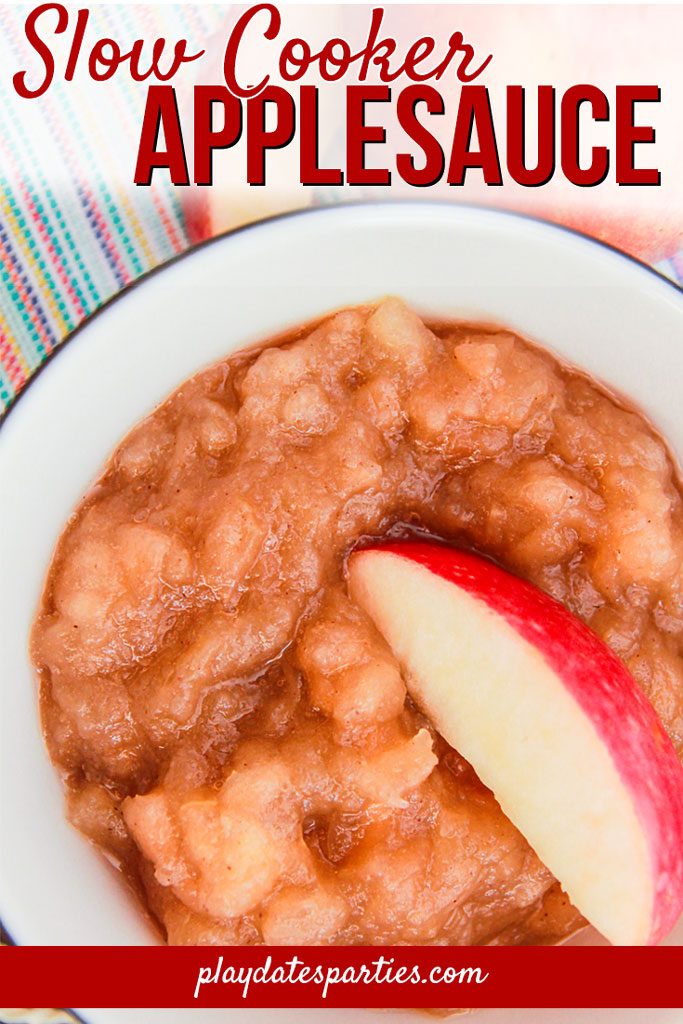This image showcases a vibrant and inviting cover of a cookbook titled "Slow Cooker Applesauce." At the top of the cover, the title is prominently displayed with 'Slow Cooker' written in a cursive red font, left-aligned, and 'Applesauce' in larger, bold red letters centered beneath it. The background at the top features an eye-catching pattern of alternating vertical stripes in pink, green, white, and blue, set against a white backdrop, with a blurred faded pink and white blend on the right side.

The main section of the cover is dominated by an up-close photograph of a partially visible plate with a black rim. On the plate sits a helping of cinnamon applesauce, enriched with a brownish hue and a wedge-shaped slice of apple with red peel nestled on top, hinting at freshness and flavor. This plate appears to be placed on a colorful kitchen towel, adorned with stripes in green, blue, red, yellow, and white.

At the bottom of the cover, a red rectangular banner with white letters prominently displays the source, "playdatesparties.com," adding a final touch to this visually appealing and taste-provoking cookbook cover.